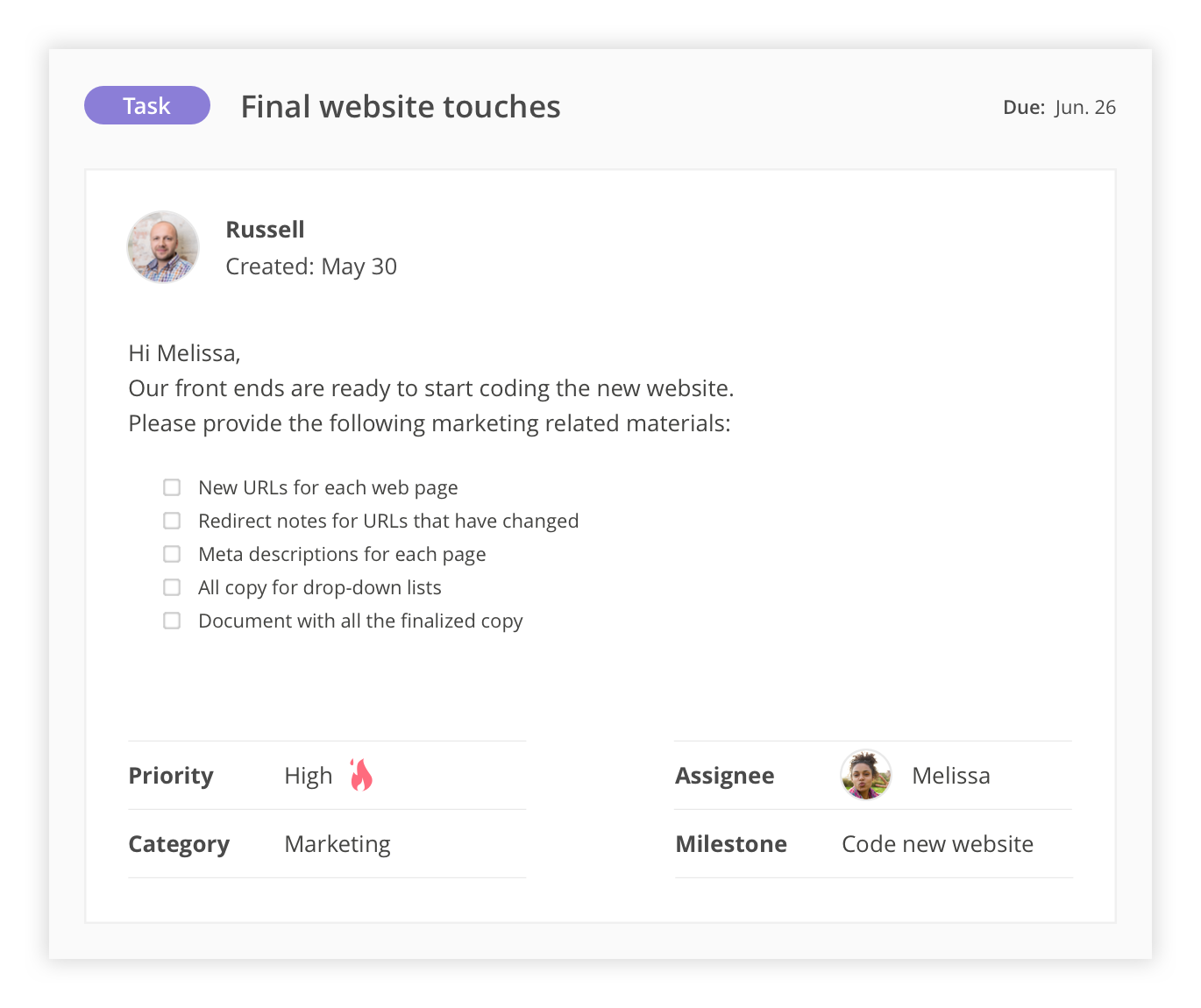In the image, there is a square with an off-white background. In the upper left-hand corner, a purple oval contains the white, capitalized letters "TAS". Adjacent to this, in black text, it reads "Final Website Touches" with the "F" in "Final" capitalized. On the right-hand side, there are the words "Do," followed by an ellipsis and "Jun. 26".

Within the shape, there is a white rectangle containing a circular profile picture of a man wearing a plaid shirt, identified as Russ. The text alongside him reads "created... May 30th". Below this, the text begins with "Hi, Melissa," followed by "Our front ends are ready to start coding the website. Please provide the following marketing-related materials:"

Then, there are five bullet points each outlined in gray:
1. New URLs for each webpage
2. Redirect notes for URLs that have changed
3. Meta descriptions for each page
4. All copy for the dropdown list
5. Document or finalized copy

Following the list, in black text, it states "Priority: High" with a red flame icon, and "Category: Marketing". Finally, on the other side, it says "Assignee: Melissa" and "Milestone: Code new website".